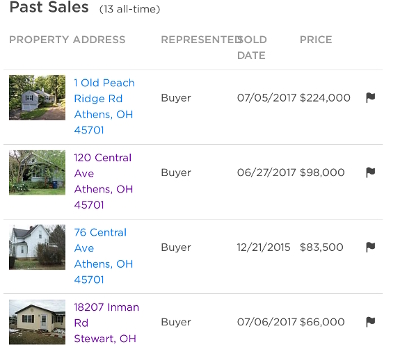Here is a detailed and cleaned-up caption for the image:

---

Screenshot of Sold Properties

Displayed at the top left of the image are the words "Past Sales" in black, capitalized text, followed by "(13 all-time)" in parentheses. Below this header, the information is organized into columns titled "Property Address," "Represented," "Sold Date," and "Price." These column titles are all in gray, capital letters.

Under "Property Address," there are four rows, each featuring a small square image next to the property's address. The addresses alternate in color between blue and purple text. 

1. The first property is listed as "10 Peach Ridge Road, Athens, Ohio, 45701" in blue text.
2. The second property address is in purple text.
3. The third property address is back in blue text.
4. The fourth property address is again in purple text.

For the "Represented" column, each property is marked as "Buyer."

The "Sold Date" column lists the following dates for each property:
1. 07-05-2017
2. 06-27-2017
3. 12-21-2015
4. 07-06-2017

In the "Price" column, the sale prices are recorded as:
1. $224,000
2. $98,000
3. $83,500
4. $66,000

Each entry has a black flag icon next to it.

---

This caption accurately describes the elements in the screenshot of sold properties in a detailed and structured manner.